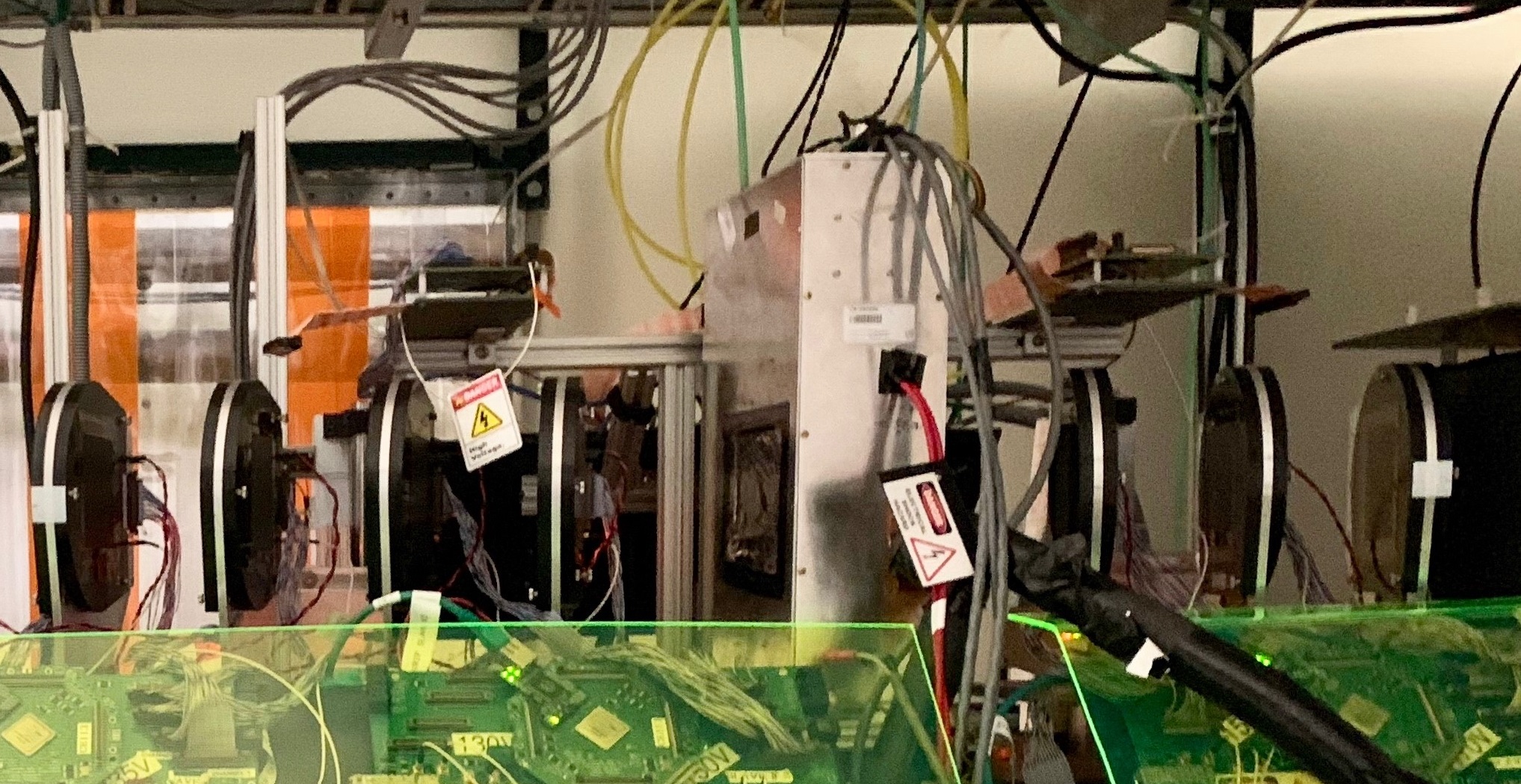This grainy photograph captures a detailed view of a technical setup, likely related to a scientific experiment or industrial machinery involving computer components. The background features a white wall adorned with a series of vertically mounted black circular disks, each spaced about half a foot apart. These disks, characterized by a silvery stripe down their centers, have various wires and cables extending from the tops and backs, connecting to other equipment and disappearing into the ceiling.

Prominently in the center, there is a large light metal apparatus or box equipped with multiple cables, including yellow, green, and black ones coiled and hanging down. A caution logo and warning sign mark this box, which also bears a label with a barcode. Red cables with a danger sign extend from this apparatus.

To the left and right, more circular disks are attached to white posts, maintaining the same configuration. Gray accordion tubes hang vertically on the left side of the frame. In front of this entire setup, a neon green translucent pane of plastic spans the lower quarter of the image, offering a view of numerous circuit boards and computer components behind it. These boards are densely populated with connections, as various cords extend in and out, further illustrating the complex and interconnected nature of the equipment. The setup overall gives the impression of a well-organized yet intricate assemblage of technological components, indicative of a high-tech or experimental environment.